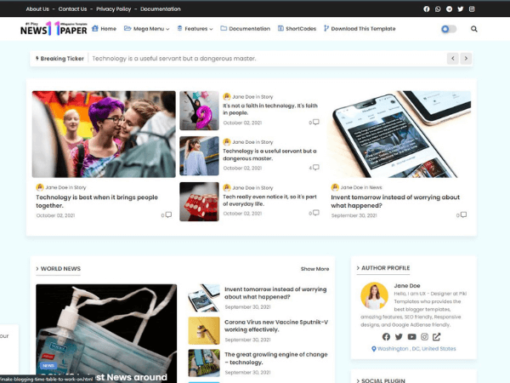This vertical screenshot captures a detailed layout of a modern webpage with several key sections and interactive elements. At the top of the image, a sleek black rectangular bar spans across the width of the screen. On the left side of this bar, white text holds navigational options such as "About Us," "Contact Us," "Privacy Policy," and "Documentation." 

On the right side of the bar, small social media icons for platforms like Facebook, Twitter, and Instagram are neatly arranged, offering quick access to these networks. Scanning back to the left, below the main bar, there's a section dedicated to navigation links, each preceding a blue icon. The links include "Home," "Mega Menu," "Features," "Documentation," "Shortcodes," and "Download This Template." A toggle switch and a magnifying glass icon are also present on the top right corner, likely used for settings and search functionality, respectively.

The background of the webpage has a pale bluish tint, contributing to a calming visual aesthetic. Prominently displayed is a "Breaking Ticker" with the text stating, "Technology is a useful servant but dangerous master," accompanied by left and right navigation arrows to browse through breaking news.

Below this, there are various clickable articles, each featuring an image, title, and publication date. For instance, one of the articles reads, "Technology is best when it brings people together" with the date "October 02, 2021" displayed less boldly underneath. As you scroll further, more sections appear, including one for "World News," an option to "Show More," and an "Author Profile" section showcasing an author’s picture, name, and a brief description, with an option to click for more information.

Overall, this detailed snapshot effectively summarizes a webpage designed for easy navigation and engagement, featuring a blend of visual and textual elements curated for a dynamic user experience.